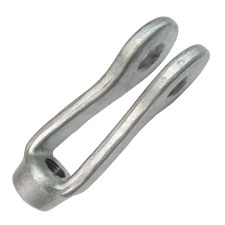The image features a small, intricate piece of silver metal against a white or transparent background. The object has a rounded base tilted towards the bottom left of the image, from which two identical arm-like extensions rise upwards and to the right. These arms form a narrow horseshoe shape, each with holes perfectly aligned at their opposite ends, resembling spoons with perforations. The base suggests it can be screwed or tightly fitted into place, making it potentially useful for stringing or hinging purposes. The metal appears to be stainless steel.